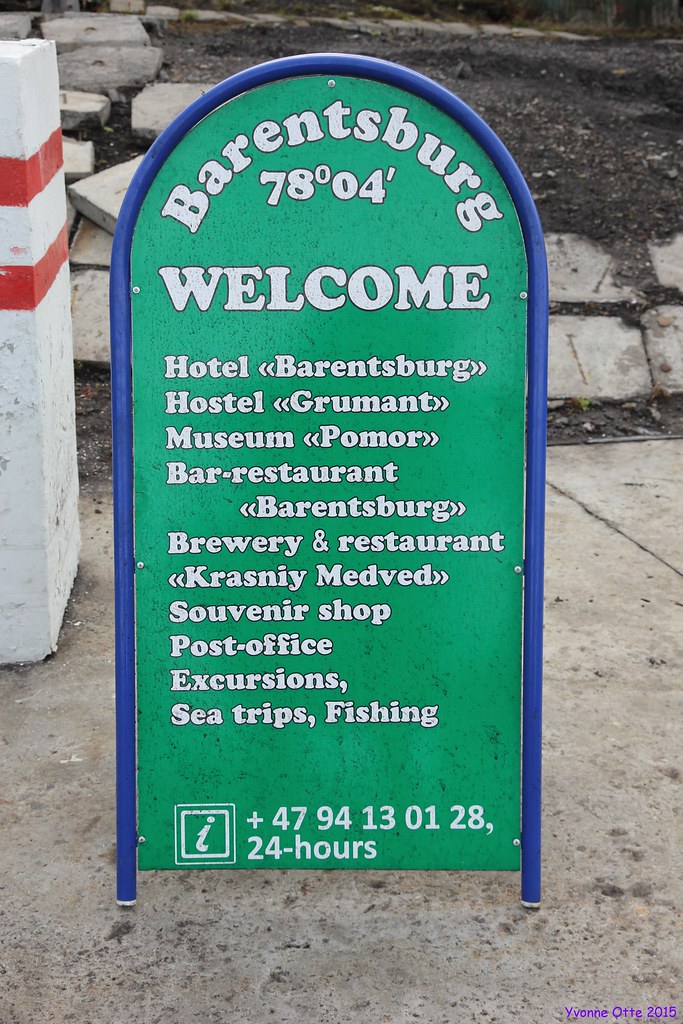This is an image of a tall, metal directional and informational sign placed on a sidewalk near a garden bed. The sign has a distinctive blue, dome-shaped border, resembling a bullet, and features a green background with white text. At the top of the sign, it reads "Barentsburg 78°04'" and "Welcome". Below, the sign lists several locations and services: "Hotel Barentsburg, Hostel Grumont, Museum Pomor, Bar-Restaurant Barentsburg, Brewery and Restaurant, Krasny Medved, Souvenir Shop, Post Office, Excursions, Sea Trips, Fishing." At the bottom, there is an information icon with a phone number, "+47 94 13 01 28," indicating 24-hour availability, and a small white post with red stripes is visible on the left side of the image.